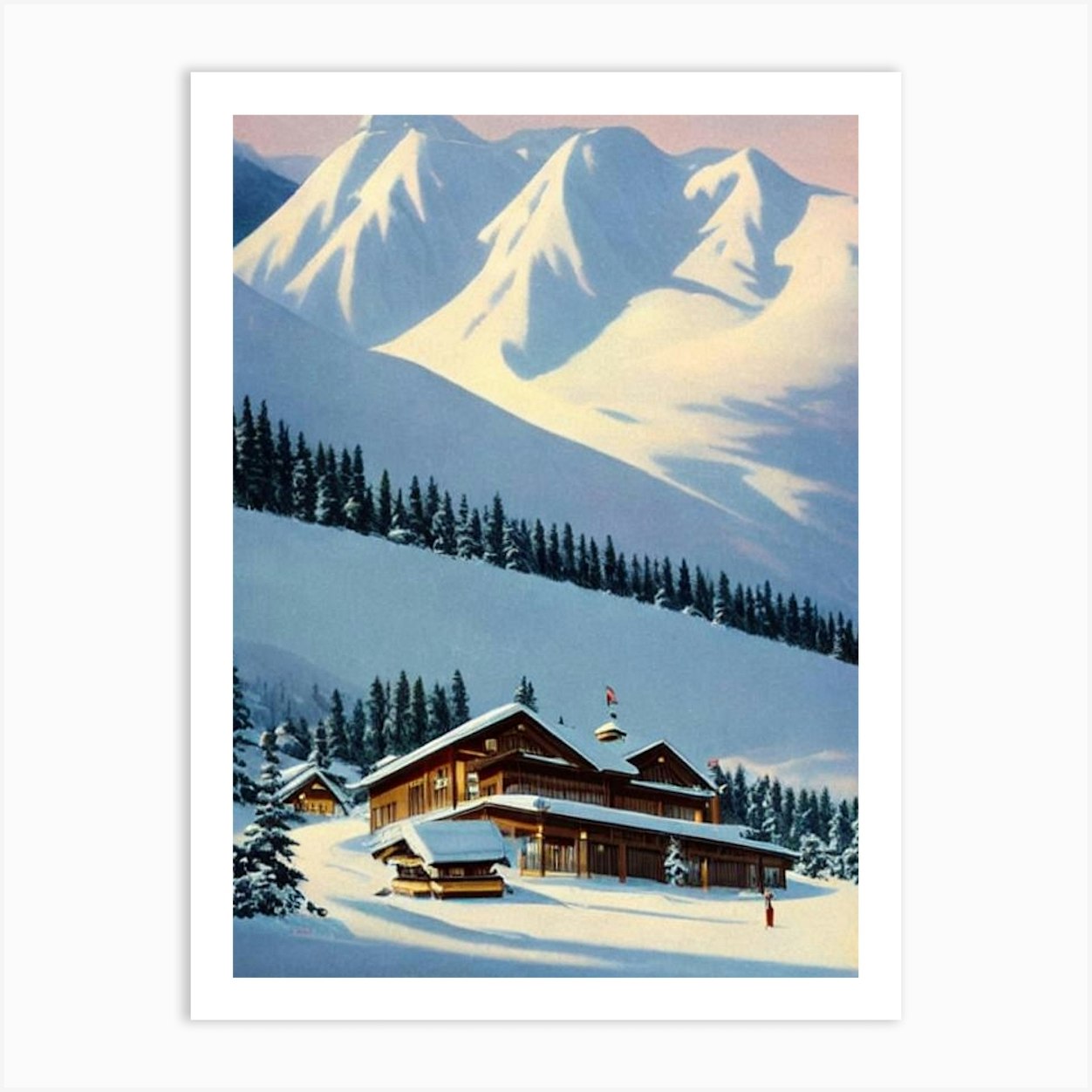This print is reminiscent of the iconic National Parks posters created by the Works Progress Administration. It captures a serene wintry landscape. At the top, towering, snow-covered mountains dominate the scene, their icy peaks standing majestically. Midway down the image, a dense forest of pine trees stretches horizontally across the panel, adding a touch of evergreen life to the frosty environment. At the base of the print, a quaint ski lodge or mountain cabin is nestled among the trees, its roof blanketed in thick snow. Surrounding the main structure are several smaller buildings, all similarly adorned with snow. The print, rendered in a portrait orientation, is bordered with a pristine white matting, further enhancing its classic and timeless appeal.